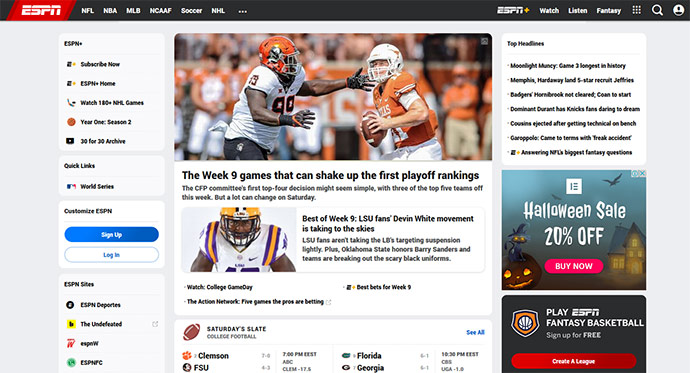On the ESPN website, the vibrant red ESPN logo is prominently displayed at the top within a red square, featuring the letters "ESPN" in white. Below the logo is a horizontal black navigation bar with headings for different sports categories such as NFL, NBA, MLB, NCAAF, Soccer, and NHL, all written in white. To the right of these headings, additional options like "Watch," "Listen," and "Fantasy" are provided, along with icons for search (magnifying glass) and user accounts (people icon).

The focal point of the image is a dynamic football scene set against an orange-dominated background. Two football players are prominently featured, both dressed in the team colors of orange and white. One player sports an orange helmet and orange jersey, while the other is in a white jersey with an orange helmet. This particular segment highlights a headline about a pivotal Week 9 game poised to influence the initial playoff rankings, along with a feature on LSU's Devon White demonstrating exceptional athletic movements.

Additionally, the site includes an advertisement for a Halloween sale offering 20% off, depicted with festive imagery of a pumpkin and a cat wearing a hat. Below the advertisement is a prompt encouraging users to play ESPN Fantasy Basketball, with options to sign up for free and create a league.

The lower section of the site showcases a variety of elements such as top headlines, customization options for the ESPN website, and user account actions including sign-up and login prompts. Here, users have a myriad of categories and options to enhance their experience on the ESPN platform.